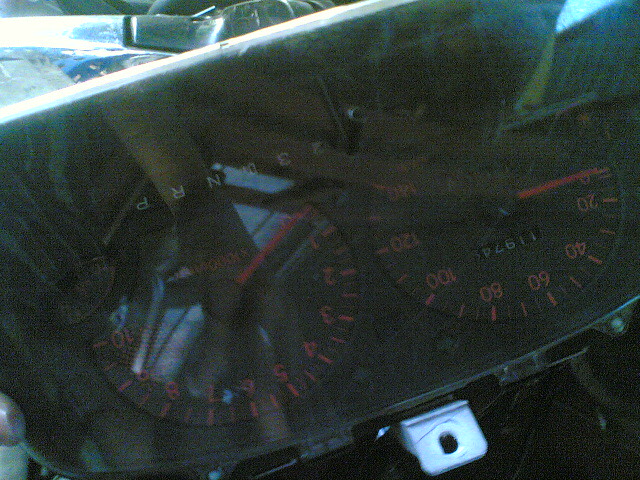A close-up photograph depicts a vintage speedometer, likely removed from its original vehicle. The speedometer appears to be upside down and angled slightly downward to the left, hinting that it has been detached and is not in its natural position. A noticeable metal bar with a screw hole is visible at the top, further suggesting it was once secured in a dashboard. The image is zoomed in or cropped, making the background indistinct and difficult to identify.

The speedometer features a distinctive design with red text and numbers on a black background. The gauge displays mileage, with an odometer showing approximately 119,000 miles. Positioned at the bottom are symbols indicating different gears (PRND), commonly found in vehicles to help drivers determine their gear selection. A black bar, likely used for resetting the mileage, is also visible at the bottom when the speedometer is oriented correctly. The overall layout and design of the speedometer hint at it being from an older model vehicle or motorcycle, adding a touch of nostalgia to the photograph.